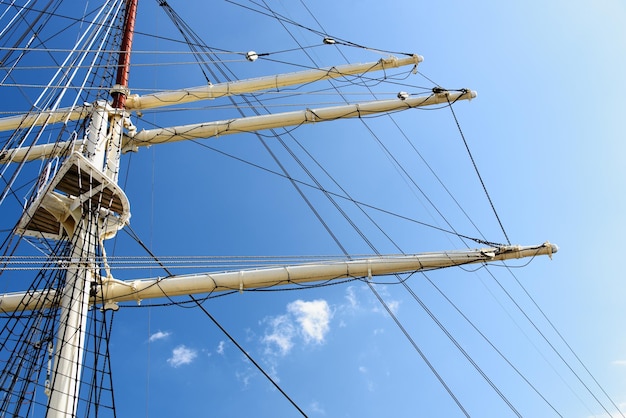This image is a close-up, landscape-mode photograph focusing on the mast of a large ship. The shot is taken from the deck looking upward into a bright blue sky with some thin, spotty clouds. Dominating the central part of the image is a tall, vertical mast that starts white at the bottom and turns rusty orange or darker brown at the top. Attached to the mast are three horizontal crossbars, which are beige-colored, and numerous black rigging lines stretched outward both vertically and horizontally. Some lines appear as rigged netting, possibly for climbing, leading up to what might be a crow's nest. The overall composition highlights the intricate details of the sail and rigging against a sunlit, clear sky, creating a vibrant maritime scene.